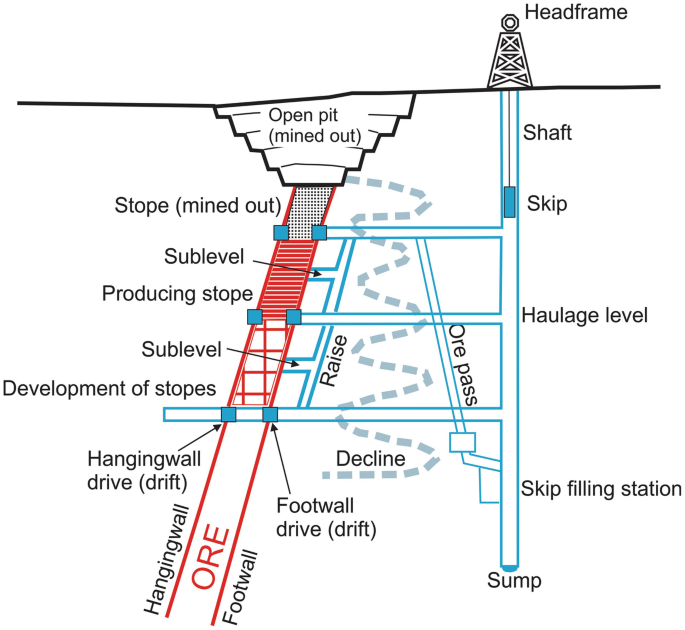This detailed diagram illustrates an underground mining operation. At the top portion of the diagram, a black horizontal line represents the Earth's surface, topped by an edifice labeled "headframe," which resembles an oil derrick. Beneath this line extends a vertical shaft, depicted with blue and red pipes. The main vertical shaft is linked to multiple horizontal shafts: a haulage level in the middle, an unmarked shaft above it, and another unmarked one below. 

To the left, a larger vertical red pipe connects these horizontal shafts. Each component of the mining system is meticulously labeled – from the shaft, the skip, the haulage level, to the skip filling station, sump, and ore pass. The diagram also shows a cross-sectional view of the Earth's subsurface, detailing various mining zones. 

At the top is an area marked "open pit (mined out)," beneath which lies a "stope (mined out)." Diagonally descending from the open pit is an ore body. Successive layers illustrate different stages of ore extraction: a "producing stope," labeled with a red dashed area, and a "developing stopes" area beneath that.

Additionally, there are two blue boxes at the depth corresponding to the lowest horizontal shaft, named "hanging wall drive (drift)" and "footwall drive (drift)." These indicate the upper and lower sides of the slanted ore body, known as the hanging wall and footwall, respectively. The comprehensive layout also highlights excavation terms and stages such as sublevel, raise, decline, and various development and operational stopes, leading ultimately to ore extraction.